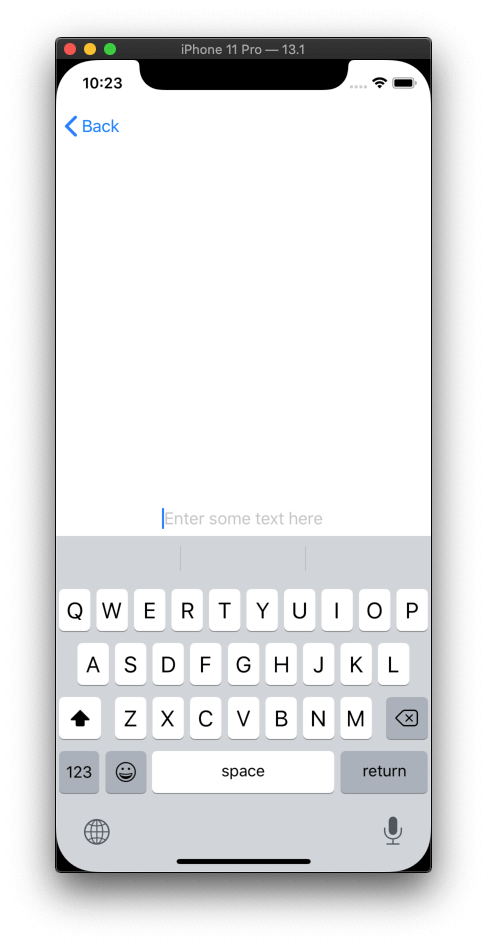This is a highly detailed screenshot of an iPhone 11 Pro running on iOS 13.1. At the very top center of the screen, it displays a black bar labeled "iPhone 11 Pro - 13.1". To the left of this label, three small colored dots are visible: red, yellow, and green. Below this, approximately half of the screen is blank white space, with the digital time "10:23" displayed prominently in black text on the upper right corner, alongside symbols indicating full internet connectivity and battery charge.

On the upper left, there is a blue-colored caret pointing to the left, accompanied by the word "Back". The rest of the display remains blank until about halfway down the screen where the prompt "Enter some text here" is situated above a blue bar. Below this section, a standard digital keyboard with a light gray background is visible.

The keyboard layout is typical for an iPhone, featuring the keys Q, W, E, R, T, Y, U, I, O, P on the top row. The keys A, S, D, F, G, H, J, K, L appear on the second row. The third row contains a shift arrow, the keys Z, X, C, V, B, N, M, and a backspace key represented by an arrow pointing left that is enclosed in a square with pointed edges.

Below these keys, on a final row, the keyboard includes a button labeled "123" for switching to numerical and special characters, a smiley face symbol for accessing emojis, and a long spacebar. Additionally, there are a return key to the right, and to the left, symbols for the globe indicating language selection and a microphone for voice input.